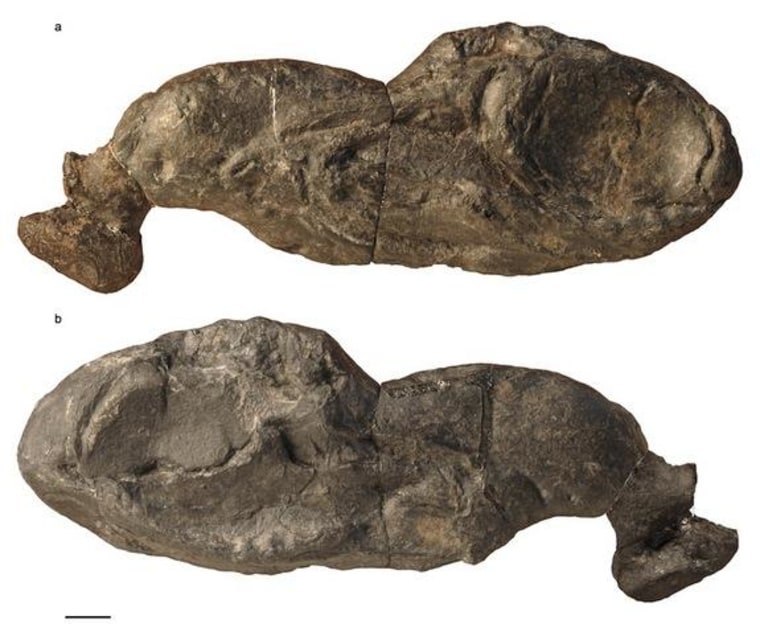This image depicts two small, prehistoric fossilized shark remains, labeled A and B, arranged vertically with the top fossil oriented right to left and the bottom oriented left to right. Both fossils are brown and show visible cracks, indicating their age and fragility. Fossil B reveals primitive fin structures near the head, though details are not very clear due to their antiquity. The shapes of the fossils resemble deflated balloons, with tapered ends that give them a somewhat foot-like appearance. The surface of the fossils features rock formations, adding to their stone-like texture. A thin black line separates the two fossils, enhancing the details of these ancient specimens.